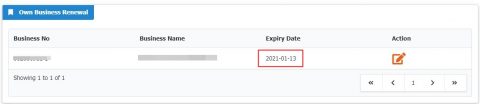This image appears to be a heavily cropped and low-quality screenshot of a section from an application or webpage, presented in a rectangular format. The rectangle is outlined by a faint gray border, visible on all sides. In the upper left corner, there is a blue rectangular box featuring a white icon on the left side and some white text, although the details of the text are unclear due to the image quality. Below this blue box, there is a section with header labels aligned horizontally from left to right, which read "Business Number," "Business Name," "Expiry Date," and "Action." The specific details of the "Business Number" and "Business Name" fields have been intentionally blurred. The "Expiry Date" field clearly displays "13th January 2021." Directly under the "Action" label is a pencil icon, indicating an editable function.